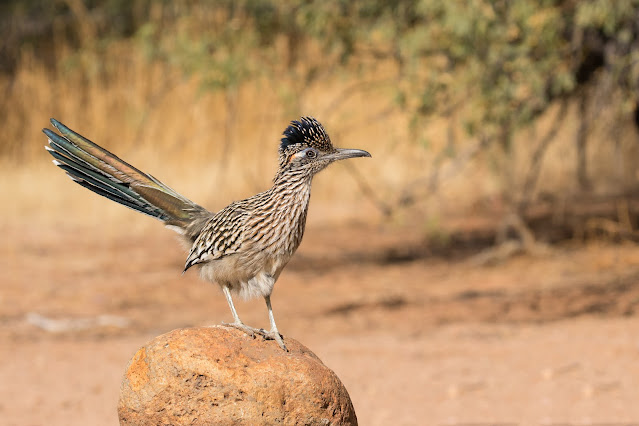The high-resolution photo captures a striking image of a small bird perched on a large, light brown boulder in an arid, sandy environment. The boulder itself has a yellowish-brown hue, and the background features muted greens and yellows from sparse trees and weeds. The ground is a sandy light brown, characteristic of dry landscapes which could be reminiscent of areas in Africa.

The bird's feathers are a complex mix, giving an overall striped pattern of off-white and black, mingled with various shades of brown and light brown. Notably, the bird sports a distinctive crown of black feathers interspersed with light orange stripes, creating a mohawk-like appearance. Its face is a grayish white adorned with a yellow-orange streak that highlights its small black eye. The bird's long silvery beak contrasts with its compact size.

Adding to its unique appearance, the bird's legs are white, and its tail feathers exhibit a blend of black, brown, and light orange. The bird's wings continue the color theme with brown and light brown feathers, making it an exquisite subject in this arid, tranquil setting.